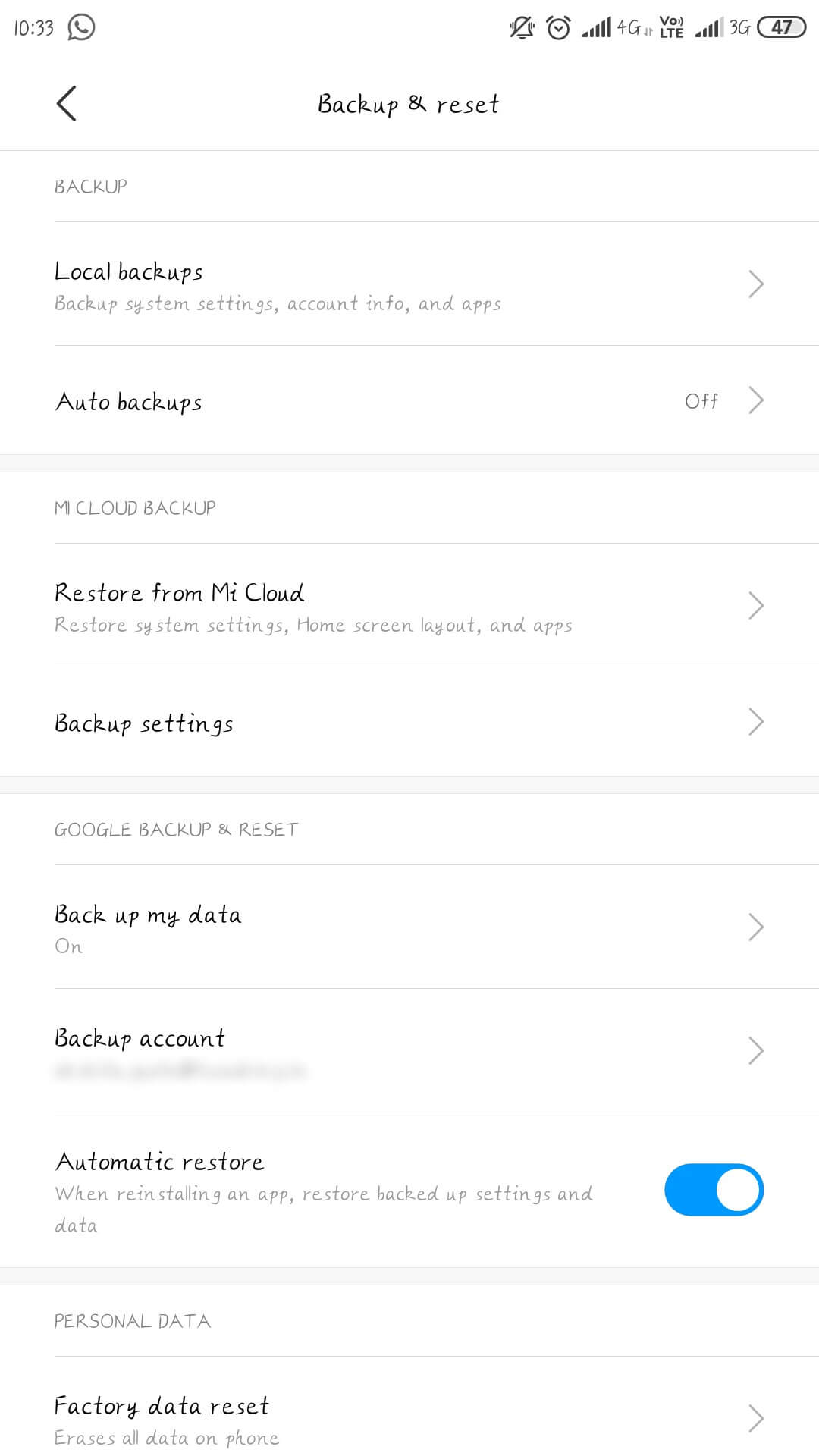This image appears to be a screenshot taken from a smartphone. In the top left corner, the time is displayed as 10:33, accompanied by a phone icon. On the top right, there is a bell icon with a line through it, indicating the phone is on silent mode, followed by a clock icon and a fully filled signal bar. Adjacent to that, the acronym "LTE" is shown next to another signal bar that is almost full, missing just one bar, followed by "3G". 

Further along, a number "47" is visible inside an oval button. Centrally located below this section, the text "Backup & reset" is prominently displayed with an arrow pointing to the left underneath a thin separating line. 

Subsequently, the options "Local backups" and "Auto backups" are listed, each with an arrow pointing to the right, divided by another gray line. Following these, the section titled "Cloud backup" features two options: "Restore from Mi Cloud" and "Mi Cloud backup settings," both indicated with arrows pointing to the right.

The next section headers "Google Backup and reset" and includes options such as "Backup my data," "Backup account," and "Automatic restore." The "Automatic restore" option is accompanied by a toggle switch on the right, which is currently turned on. Towards the bottom, under the section labelled "Personal data," the option "Factory data reset" is found.

The image captures the phone's settings related to various backup and reset options with a clear and organized layout.